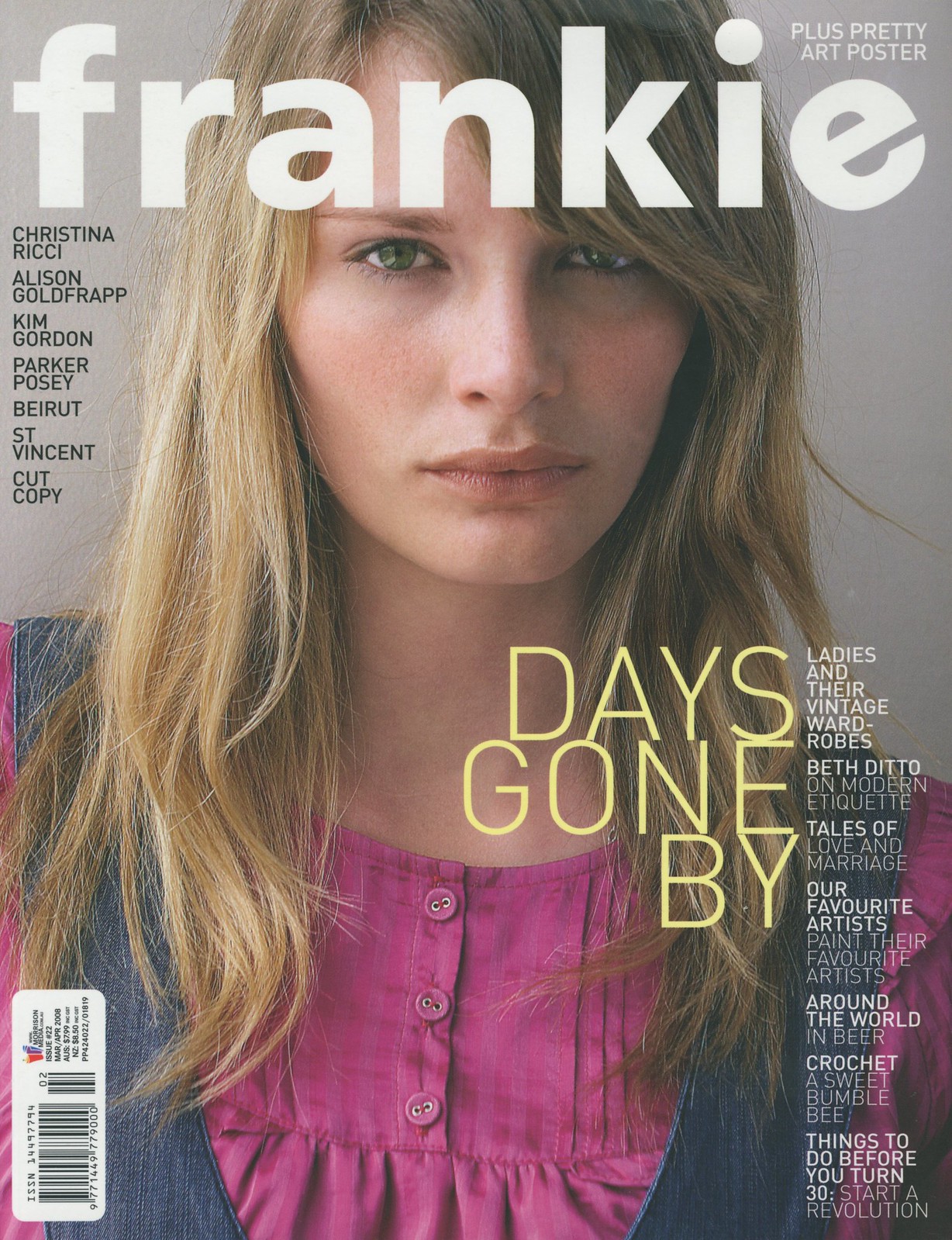The cover of the magazine prominently features the title "Frankie" in large white letters at the top. The main image is a centered photograph of a woman with long blondish hair cascading past her shoulders, wearing a blue vest over a pink shirt. She looks directly at the camera with a serious expression, her green-amber eyes deeply engaging the viewer. 

On the left-hand side, a column of names appears: Christina Ricci, Alison Goldfrapp, Kim Gordon, Parker Posey, Beirut, St. Vincent, and Cut Copy, suggesting notable contributors or features within the magazine. 

At the woman's neck level on the right side, the text "Days Gone By" is highlighted in bold yellow letters, followed by a list of intriguing article titles in smaller white text: "Ladies in Their Vintage Wardrobes," "Beth Ditto on Modern Etiquette," "Tales of Love and Marriage," "Our Favorite Artists Paint Their Favorite Artists," "Around the World in Beer," "Crochet a Sweet Bumblebee," "Things to Do Before You Turn 30," and "Start a Revolution."

The cover is vibrant with a mix of colors including blue, pink, yellow, black, white, red, purple, and gray. A barcode and some date information are positioned in the bottom left corner, emphasizing the commercial aspect of the magazine. The overall style and setting suggest a fashion-forward publication with a blend of art, culture, and personal interest stories.